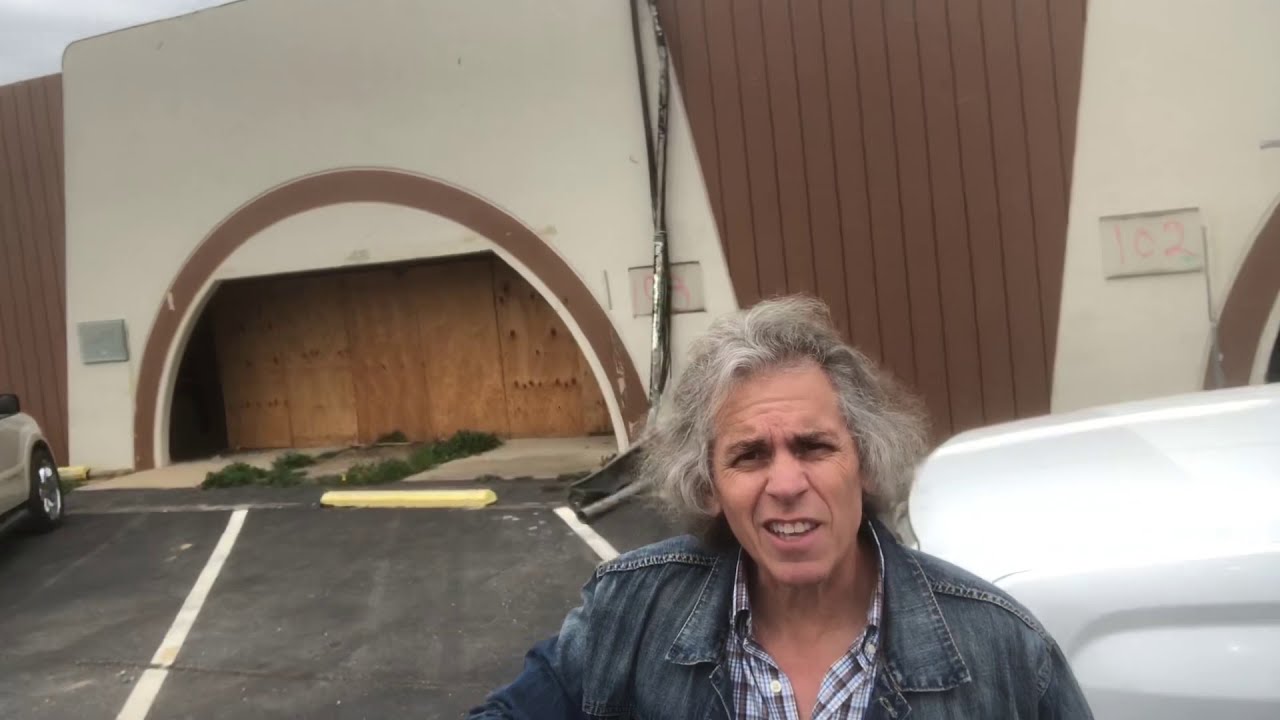In the center of the photograph stands a man making a facial expression that suggests either confusion or wincing in bright light, possibly mid-speech. He's sporting a medium blue denim jacket over a light blue buttoned-down shirt with fine black stripes and white buttons. His chin-length salt-and-pepper hair, devoid of any cosmetics, falls around his ears. Behind him stretches an older, mid-century modern or 1970s-style building with archways, boarded-up windows, and wood paneling. The structure, likely for commercial use, is flanked by parking spaces. To the man's right, there's a white car visible up to its front lights near his shoulder. A partial view of another car's front right wheel is on the photo's far left. Among the details in the background, there's a pink handwritten '102,' suggesting a parking space. The scene is further characterized by yellow parking blocks, white-striped spaces, and patches of grass.